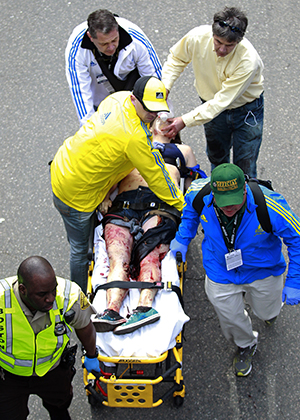The image captures a dramatic and dire emergency situation viewed from above. At the center, a severely battered and bloodied trauma victim lies on a stretcher, with their feet pointed unnaturally to the left. The individual's clothing is partially obscured but appears to include either pants or shorts and possibly some form of halter top or shirt. Surrounding the victim are five individuals actively providing assistance. 

In the forefront, a man in a yellow fluorescent vest, who appears to be a policeman or security officer, is guiding the stretcher. Beside him, another man in a blue jacket and green hat is also helping with the maneuvering. At the rear of the stretcher, one person is holding an oxygen mask over the injured individual's face, while another person is pushing the stretcher. Leaning over the victim is a third person, dressed in a yellow jacket and hat, possibly administering additional care. 

The scene is filled with urgency, and the bright colors of the helpers' clothing—predominantly yellow and blue—stand out. Most individuals on the scene appear to be casual pedestrians, possibly bystanders who have stepped in to help. The man in the yellow vest is the only African American, while the others are Caucasian.